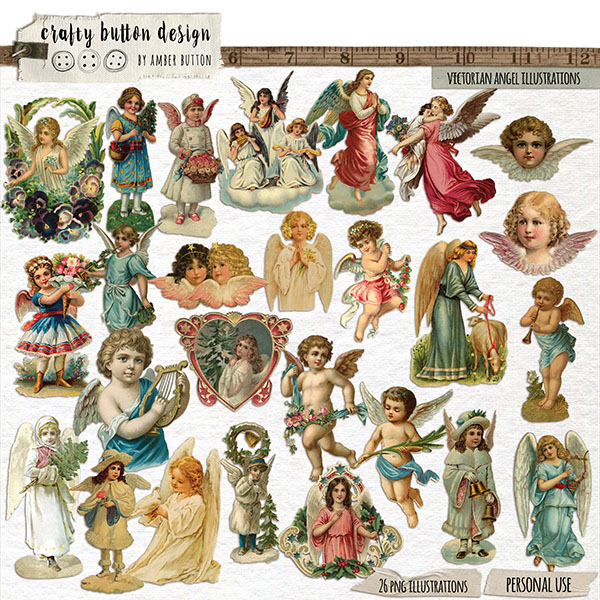This is an illustration set titled "Victorian Angel Illustrations" by Crafty Button Design, scripted by Amber Button. At the top left, a beige label with black text and three button drawings displays the brand name. To the right, a wooden ruler stretches horizontally from 0 to 12 inches, demarcating the scale. Within this frame, the top-right corner declares the set’s title. This collection comprises 26 PNG illustrations available for personal use, depicted at the bottom.

The artwork showcases a variety of youthful, cherubic angels in different poses, attired in diverse robes, and clothing of multiple colors and styles. Each angel has distinct hair colors and wings. Notably, some angels are framed within heart shapes. In the bottom section, specific illustrations include an angel dressed as a nurse, another kneeling with her wings spread, and one encircled by puppies. This detailed, multi-faceted array of angelic figures is meticulously designed for creative projects.